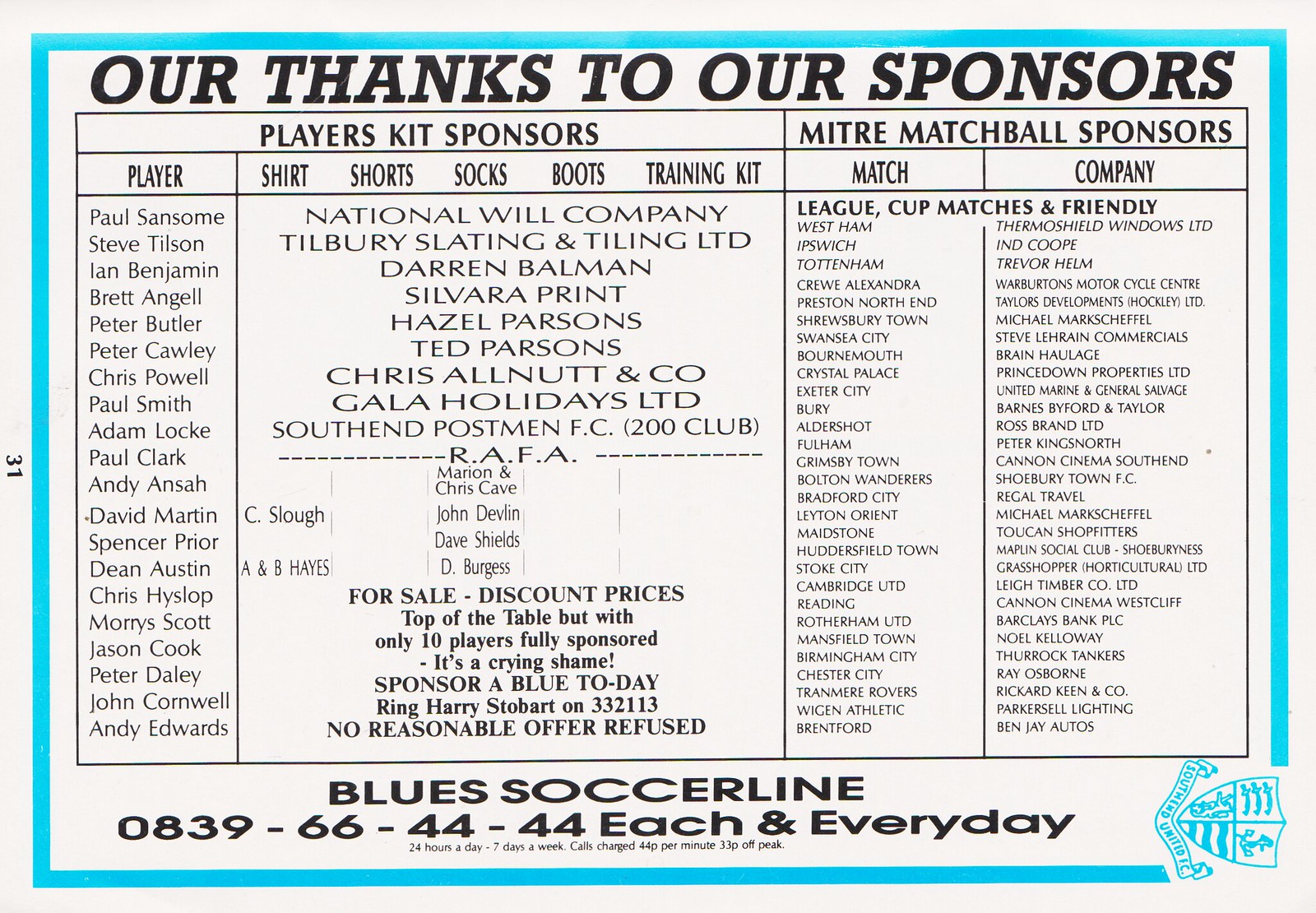The image is a flyer for a sporting event. At the top, black text reads, "Our thanks to our sponsors." Below this, the flyer is organized into several columns within black-bordered rectangles. The first rectangle reads, "Players Kit Sponsors." To the right, there is another rectangle labeled, "Meet Your Match Ball Sponsors." 

Underneath these titles, there is a detailed table listing various players and associated categories such as shorts, socks, boots, and training kits. The player's column includes names like Paul Sansom, Steve Tilson, Ian Benjamin, Brett Angell, Peter Butler, Peter Cawley, Chris Powell, Paul Smith, Adam Locke, Paul Clark, Andy Ansah, David Martin, Spencer Pryor, Dean Austin, Chris Heislop, Morris Scott, Jason Cook, Peter Daly, John Cornwell, Andy Edwards, among others. 

Additionally, it lists the sponsors for the gear and kits, including National Wheel Company, Tilbury Slating and Tilling Limited, Darren Ballman, Sylvara Print, Hazel Parsons, Ted Parsons, Chris Allnut and Co., Gala Holidays Limited, Southend Postman, FC 200 Club, and Wrappa. 

Furthermore, there is a note highlighting that only 10 players are fully sponsored and encourages readers to sponsor a player. The flyer also contains promotional details such as "For sale at discount prices, top of the table." The contact information for "Blue Soccer Line" is provided at the bottom.